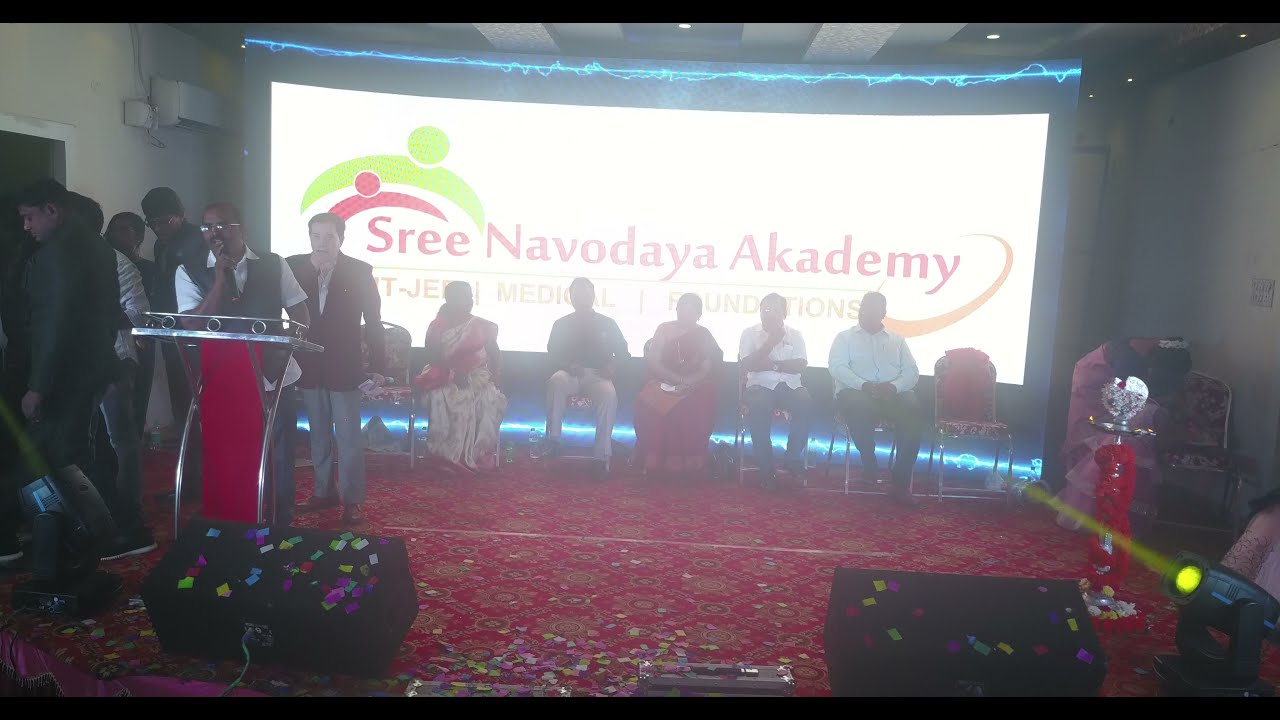The image depicts a lively event inside a building, likely a celebration or a corporate meeting, possibly hosted by Sri Navodaya Academy, as indicated by the large white screen with blue lights on top and bottom. The screen prominently displays the name “Sri Navodaya Academy” with a logo featuring children in green and red, followed by subheadings like "IIT JEE Medical Conditions." The stage is adorned in red, strewn with colorful confetti, contributing to the festive atmosphere.

In front of the screen, several people are seated; two women and three men. The women are adorned in vibrant, long, traditional Indian dresses, while the men sport semi-casual attire, including blue button-up shirts, black pants, and brown boots. They sit on an Oriental rug, positioning them in the foreground of the image.

On the left side, a man stands behind a red podium with a microphone, appearing to address the audience. He wears glasses, a vest, and a white shirt, exuding a professional demeanor. Around him, additional lights and large black speakers with colorful sticky notes are visible. Another man in a suit jacket stands adjacent to him, amid a bustling background of individuals who seem to be interacting and socializing.

In the backdrop, a lady is seen bending near a lit lamp, adding a ceremonial touch to the occasion. An exit door is also visible on the left side of the image, highlighting the indoor setting. Overall, the scene portrays a colorful and dynamic gathering, blending professional elements with cultural vibrancy.